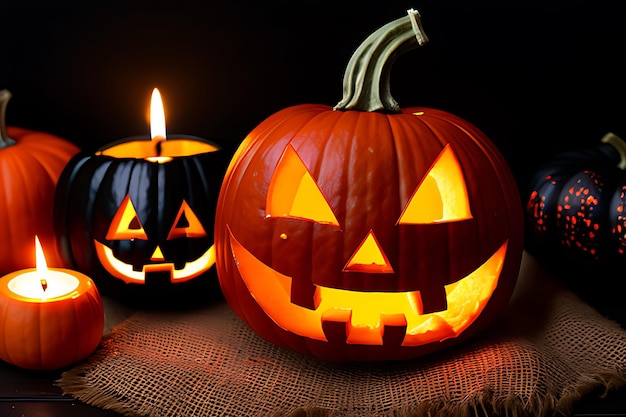This close-up photograph showcases a collection of intricately carved and uniquely decorated pumpkins, each illuminated by candles. Central in the image is a medium-sized orange pumpkin with a gray stem, featuring the classic jack-o'-lantern face: triangle eyes, a triangle nose, and a toothy, jagged grin. To its left, a black-painted pumpkin with its top removed reveals a candle flickering inside, casting a warm glow through its similarly traditional carved face. Adjacent to this black pumpkin is a small orange pumpkin holding a lit votive candle, possibly a store-bought item designed to look like a miniature jack-o'-lantern. Both the pumpkins rest on a textured burlap surface. In the background to the right, a hint of another black-painted pumpkin with distinctive orange splotches is visible, adding a striking visual contrast. The arrangement and detailed decoration of the pumpkins create a captivating, festive Halloween scene.